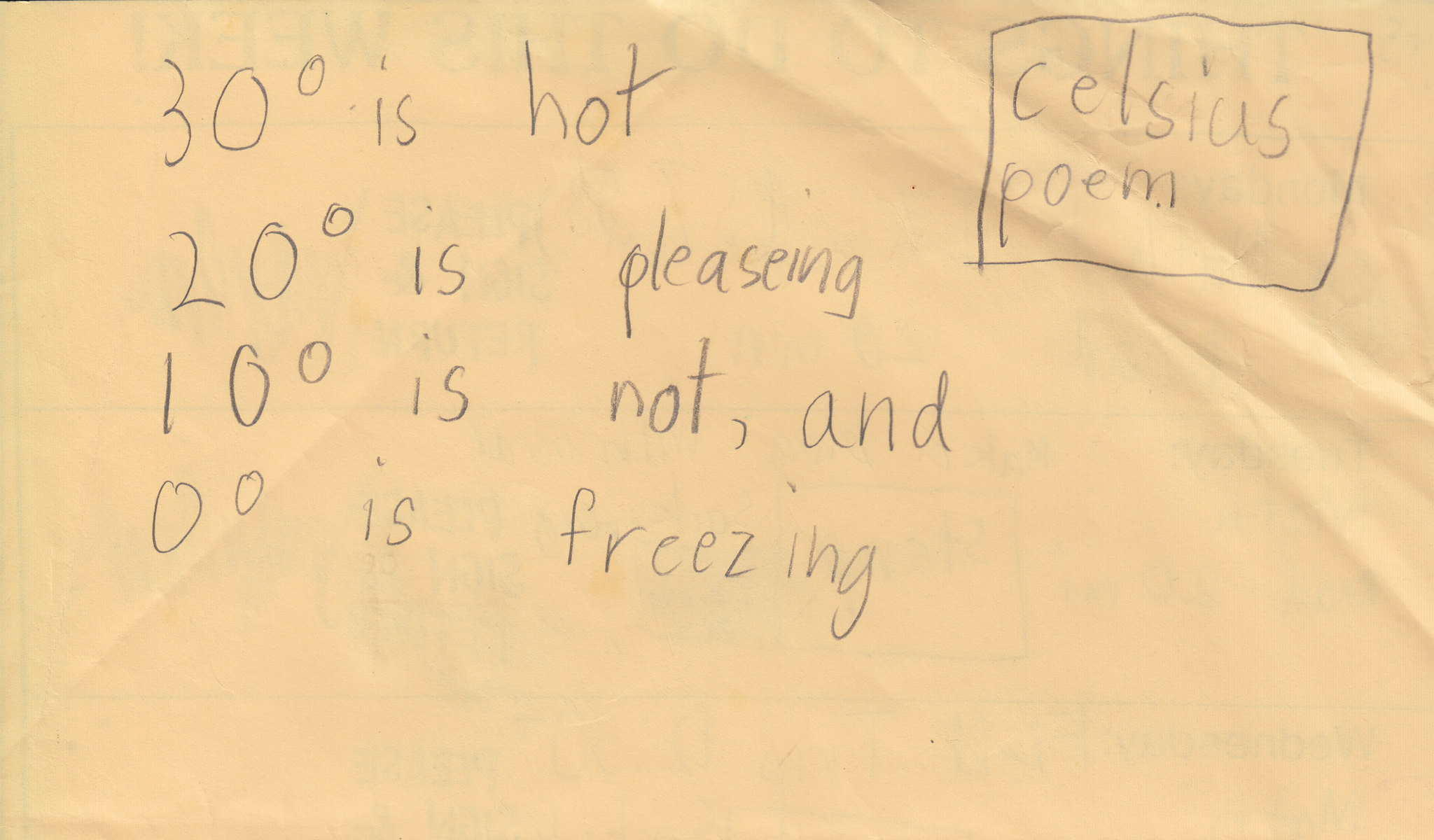This is a detailed close-up photograph of a cream-colored page, adorned with a handwritten rhyming poem in black ink, titled "Celsius Poem." The poem reads: "30 degrees is hot, 20 degrees is pleasing, 10 degrees is not, and 0 degrees is freezing." This whimsical and entertaining verse appears to be the work of a child in grade school. The title, "Celsius Poem," is enclosed within a rectangle located on the upper right side of the page. The paper shows noticeable creases, particularly at the top right corner.